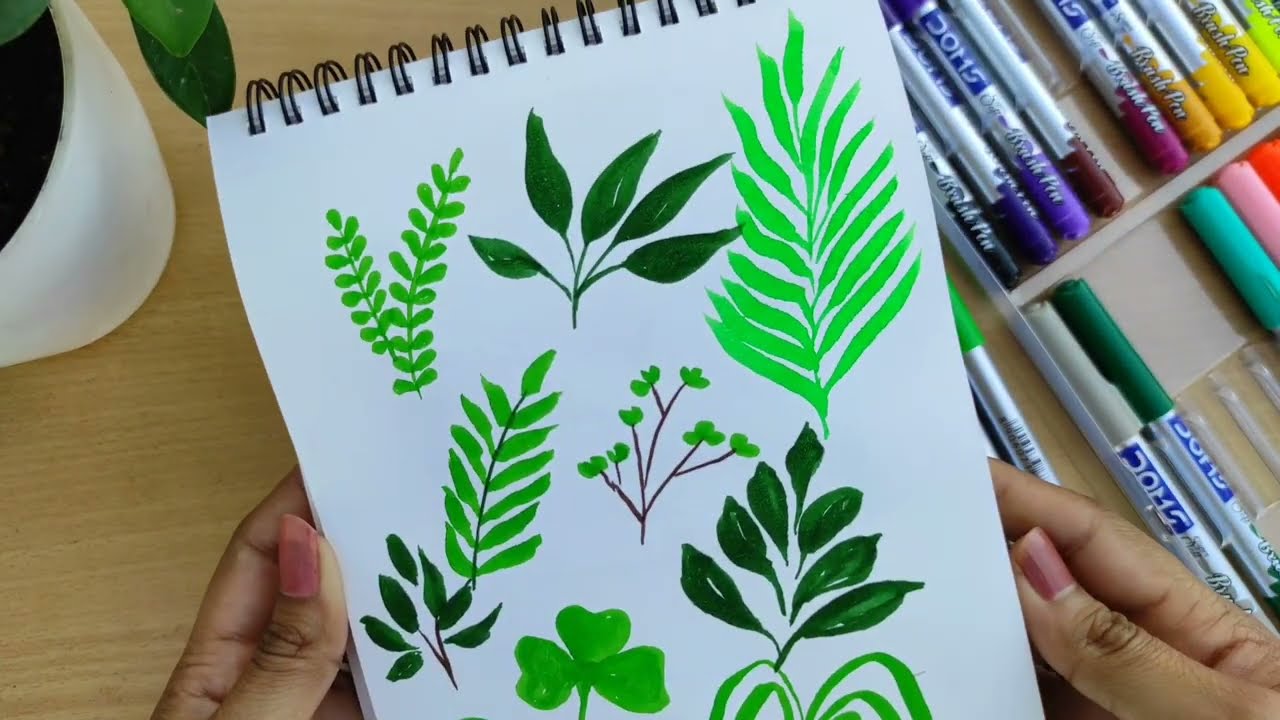In this horizontal rectangular image, a pair of female hands, adorned with light pink manicured fingernails, gracefully holds a spiral art notebook. The notebook features black spirals at the top, and the sheet of paper reveals a detailed illustration of various green leaves—some light green with long stems, others light green with short leaves, dark green with medium length leaves, and some light green with small buds at the tips. The background includes a container full of multicolored markers on the right, boasting a variety of colors such as greens, blues, reds, and yellows. To the left, partially shown in the upper corner, is a potted plant in a white pot with a few green leaves peeking out. All of this is set on a bright, light brown wooden desk, providing a warm and creative workspace backdrop.